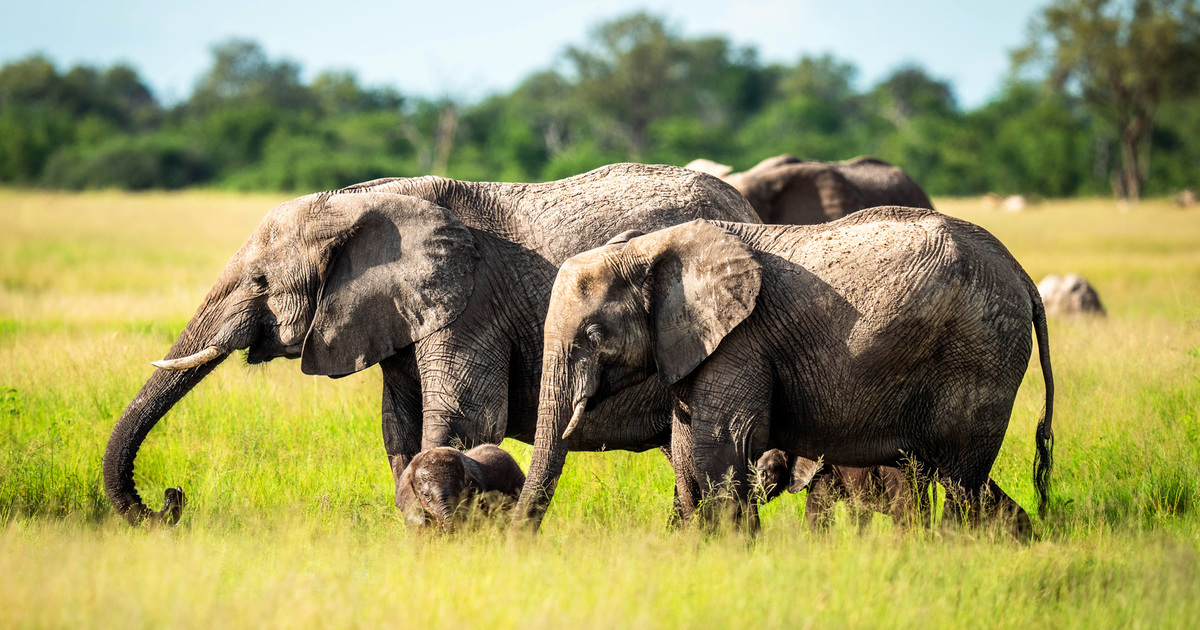A small herd of elephants is photographed traveling from the right side of the image to the left, knee-deep in light-colored tan grass. The group consists of three large elephants and two calves. The two prominent elephants in the front are adorned with tusks, with a notable size difference between them. The leading elephant, with eyes slightly open, has an elongated trunk that curves back towards the underside of its own trunk. The accompanying large elephant appears to be basking in the sunlight with closed eyes, its trunk resting on the ground. The calves stay close to the adults, sheltered under their trunks. 

In the blurred background, there is a green tree line punctuated by large stones and more grass. Further back, the greenery transitions into yellower grass. The serene composition is set against a meadow-like green grassland, drawing focus on the elephants at the front and middle of the image.